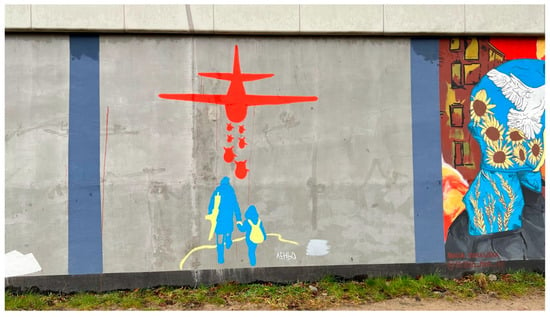The image is a horizontally oriented, color photograph of a concrete wall adorned with murals, captured outdoors with a bit of bare ground and some very low scraggly grass in the foreground. The central mural depicts a wartime scene, featuring bright blue silhouettes of an adult and a child. The adult figure is carrying a machine gun over their left shoulder and holding the left hand of the child, who is shown with a little yellow backpack. They are walking through a desolate landscape. Above them, a red silhouette of an aircraft, possibly a C-130, is depicted dropping several red bombs. There is also a yellow, squiggly line on the ground in front of them along with the artist's signature. Adjacent to this central artwork, on the right-hand side, part of another mural can be seen, showcasing the back of a woman's head with a blue kerchief adorned with a white dove of peace and some sunflowers.